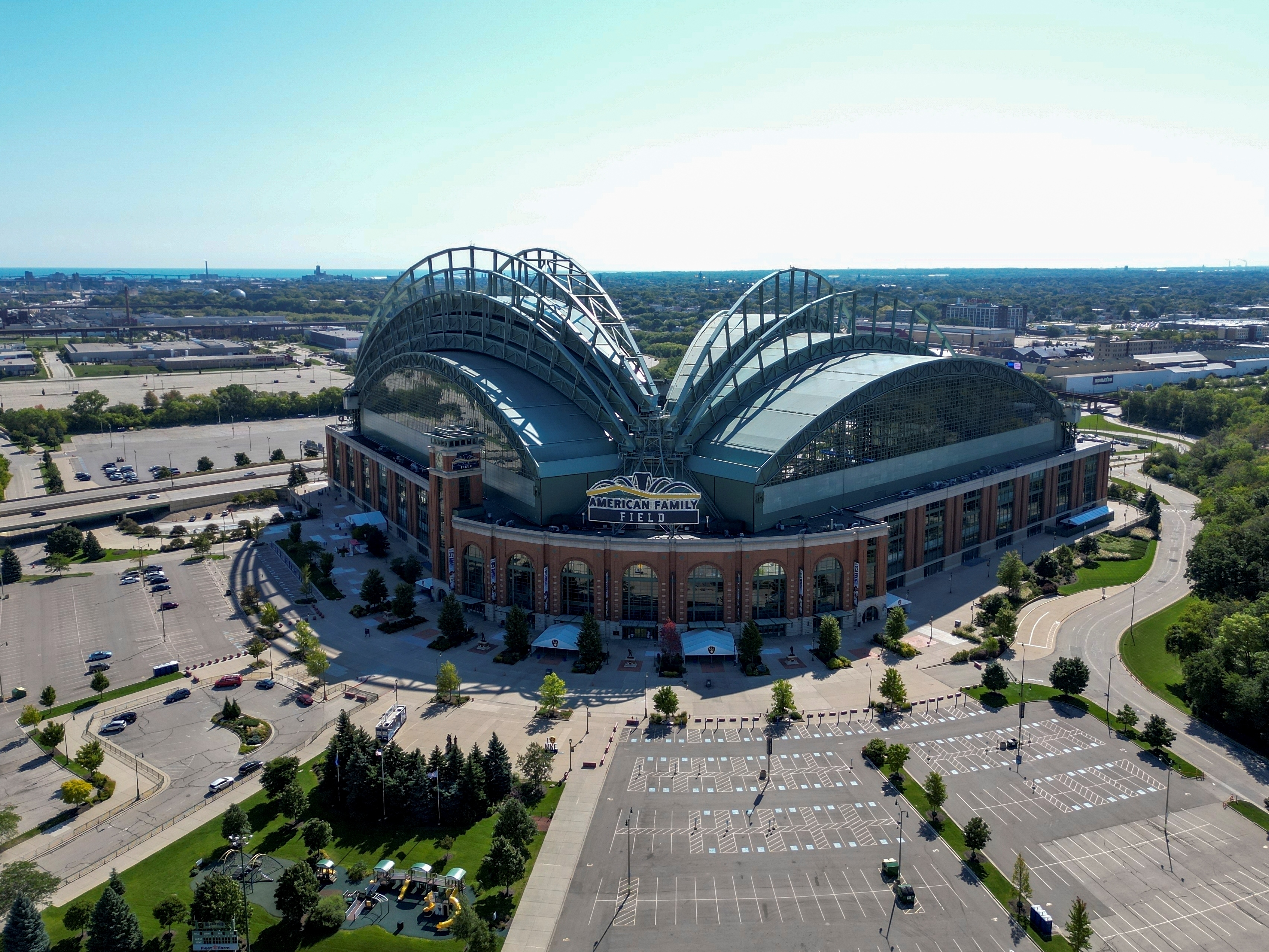This aerial image showcases a large sports arena identified by a banner that reads "American Family Field." The arena features a regular-shaped, brown-colored base with prominent, curved structures that intersect at the top, giving it a decorative and distinctive appearance. The facade of the building includes extensive brickwork, large windows, and multiple bridge-like elements enhancing its aesthetic.

Surrounding the arena is a well-manicured lot predominantly designated as a parking area. Although most parking spaces are currently unoccupied, a few cars are visible in various sections of the lot, including the left, middle, and right sides of the building. The lot is adorned with numerous trees that have green leaves and appear to be uniformly planted, contributing to the site's well-landscaped appearance.

In front of the arena, there are various entrances equipped with large white tents, providing sheltered access for attendees. A street or road flanks the right side of the building, ensuring accessible vehicular movement around the premises. The combined elements suggest this is likely a baseball stadium, especially given the open design at the back and the extensive facilities for spectators.